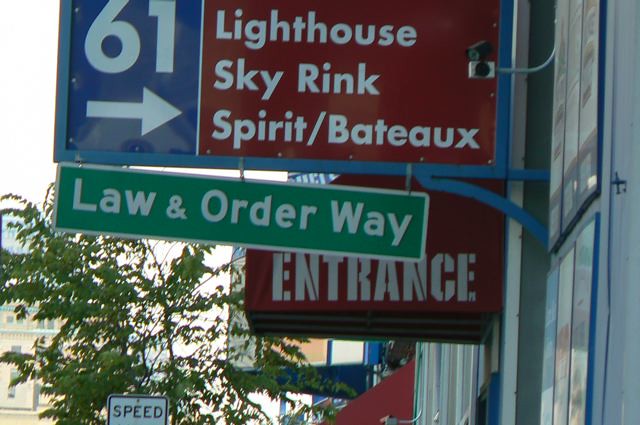The photo captures an urban downtown scene with several signs hanging outside a building. The most prominent sign in the foreground is rectangular, featuring a green and white color scheme, and reads "Law and Order Way." This sign is suspended from another sign that is colored blue and red. The upper sign indicates "61" with a rightward arrow and includes directions to "Lighthouse," "Sky Rink," "Spirit/Bateau." In the background, there's a red and white entrance sign and gray, flat-faced buildings positioned to the right. Above these buildings, a partial view of a speed limit sign is visible, displaying only the white and black colors and the word "Speed." A slender tree with green leaves stands nearby, adding a touch of nature to the urban landscape. Faint outlines of other distant buildings suggest an expansive cityscape. The brightness of the sky suggests it is a clear, sunny day.